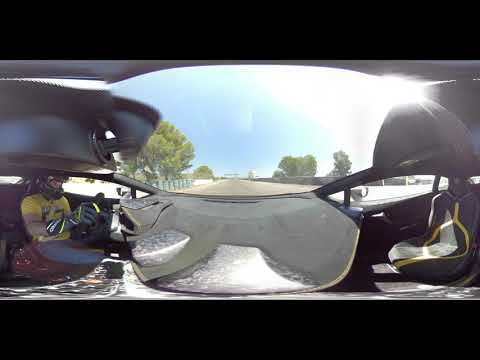This panoramic and possibly 360-degree image features a man driving a race car. The image, which seems to have been widened, provides a detailed view of the scene. On the left side, the driver is clad in a yellow t-shirt, blue jeans, thick grey gloves, and a black helmet, gripping the steering wheel. The car's interior is visible, with dark grey metal framing and a slope that curves down over the driver. A light grey dashboard spans the middle of the image, leading to the empty passenger's seat with a dark cushion on the right. Outside the windshield, the light grey pavement of the road is visible, bordered by trees under a clear blue sky with the sun shining brightly. The top and bottom of the picture are framed by thick black borders, adding to the impression that it was taken with a special panoramic or 360-degree camera. The comprehensive view includes every detail, from the car’s metal structure to the surrounding landscape, creating a dynamic and immersive scene.